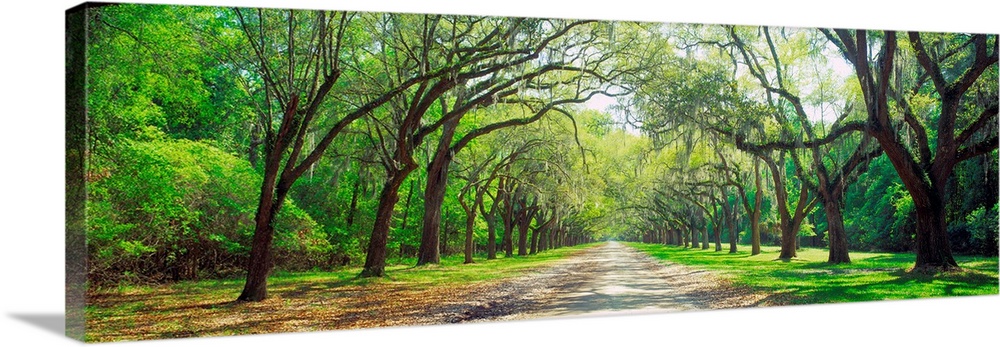The full-color photograph captures a serene outdoor scene during daylight, utilizing natural light to highlight its features. Horizontally rectangular with a bordered left side, the image resembles a small framed rectangular canvas, perfect for wall display. At the bottom center, a gray-paved road, littered with dead brown leaves, stretches vertically into the distance, framed by rows of tall, brown-trunked trees. The trees on the left have sparse green leaves and a more barren, dirt-laden ground with little grass, contrasting with the lush green grass on the right side. The trees' branches and leaves form a natural tunnel over the road, creating a canopy effect. The top portion of the photograph reveals a bright blue sky with the sun's rays shining through, adding a touch of warmth and highlighting the natural beauty of the setting. The clarity and brightness of the image emphasize the vibrant greens of the trees and grass, making the scene feel immersive and tranquil. No people, words, or numbers are present, focusing purely on the tranquil, untouched essence of nature.